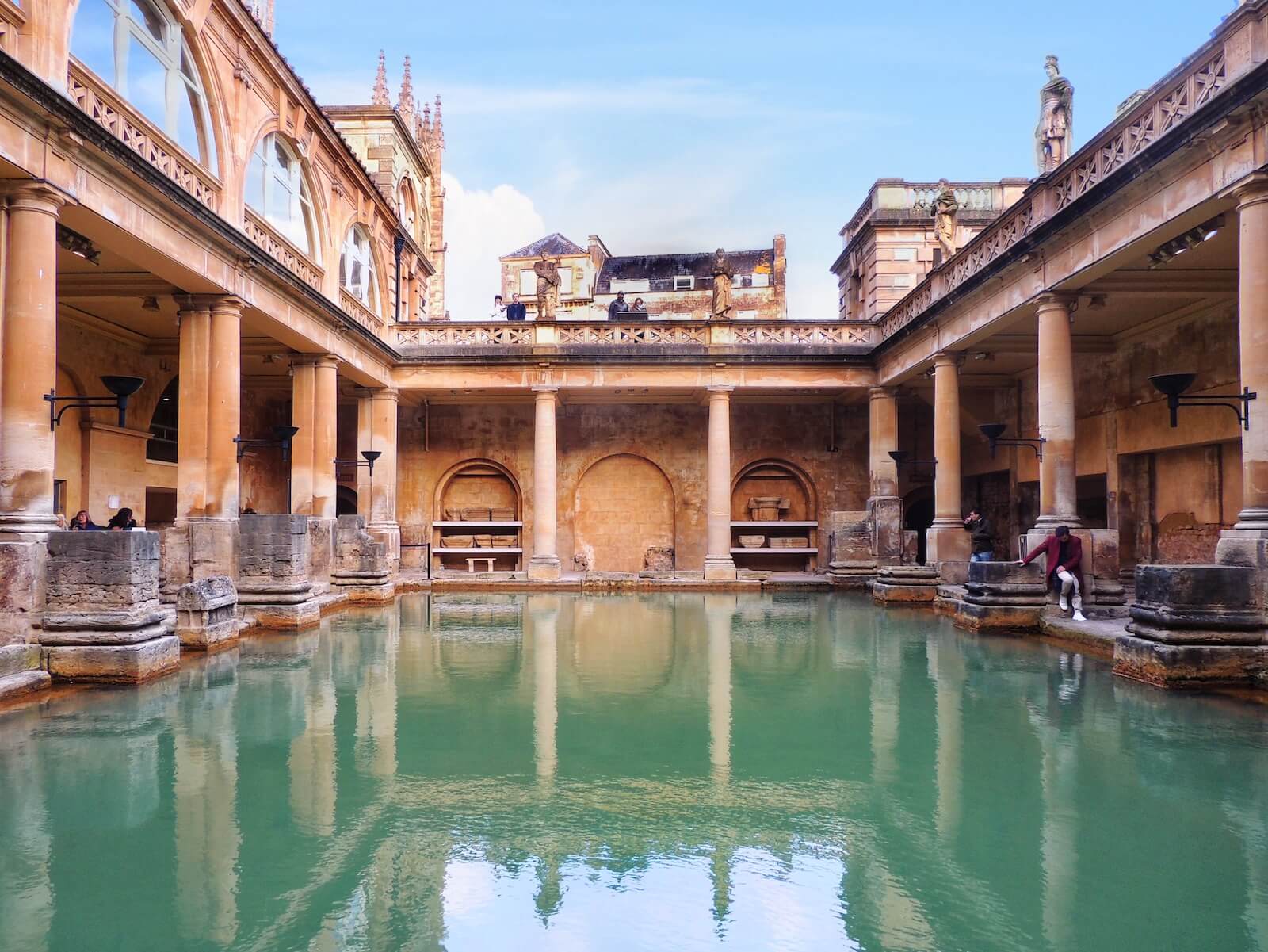A meticulously designed, luxurious building centers around a tranquil pool with striking blue water. Flanking the pool, the grand structure boasts intricate architectural details. Statues adorn the edges of the top deck, while a distinctive X or star pattern adorns the railings and outlines the rim of the roof, extending seamlessly from left to right. The backside of the building features elegant, non-functional arched designs, adding to its sophisticated appearance.

In the scene, a man clad in a red jacket, white pants, and white shoes stands prominently on the right side of the pool. Behind him, another man, dressed in a black jacket and blue jeans, appears to be talking on the phone. To the left, partially visible, are more people either sitting or standing, adding life to the serene setting.

The background showcases additional structural elements: a segment with three tall building sections capped with pointed, chimney-like features, and another smaller building with windows directly behind the pool area. On the right, yet another building sports a decorative railing, enhancing the overall ornate aesthetics. Above, the sky is a clear blue, dotted with a few white clouds, completing this picturesque and detailed panorama.